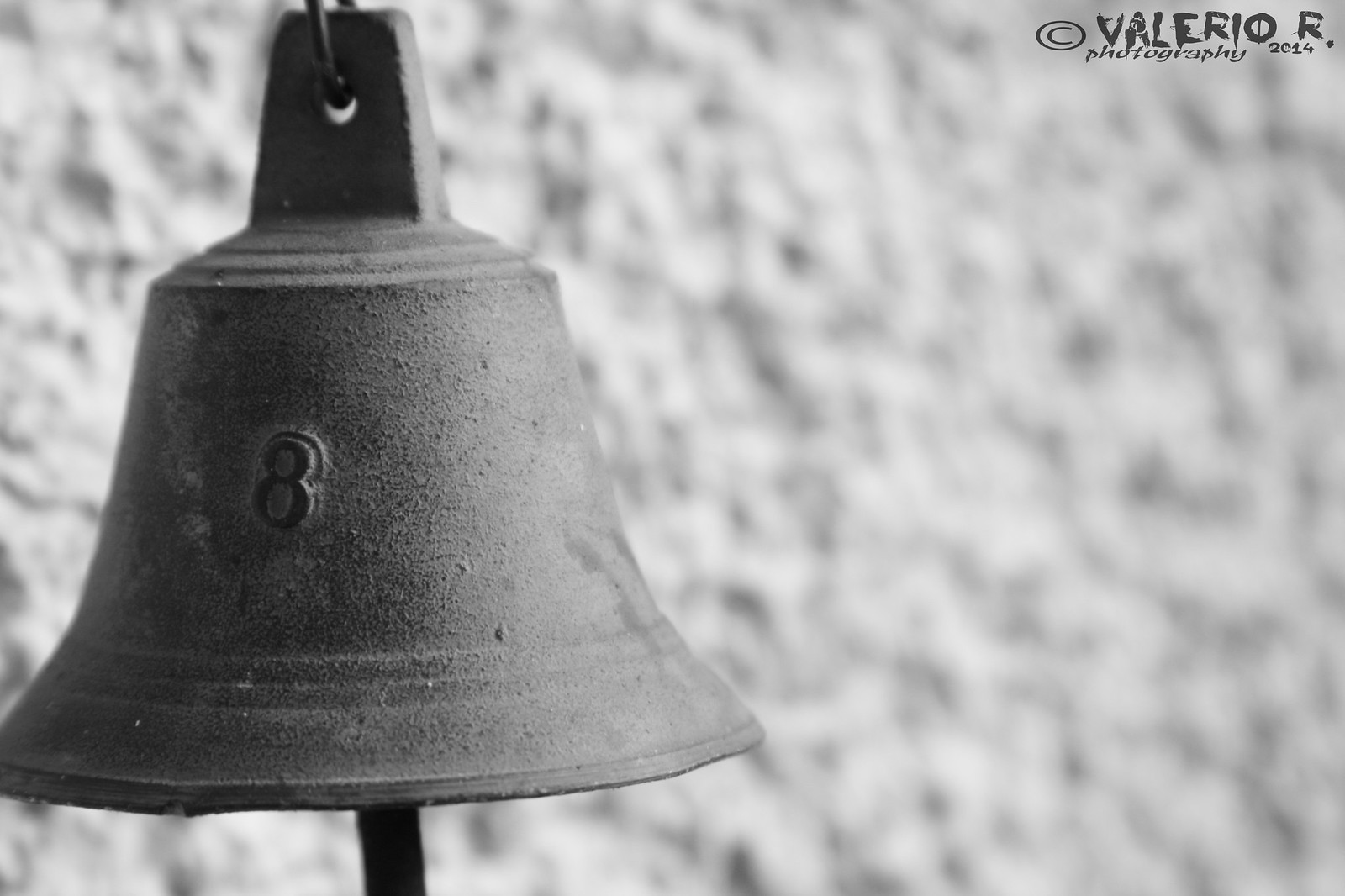This is a detailed black and white landscape photograph featuring a prominent cast iron bell in the left foreground. The bell, which has the number 8 embossed on its surface, has a slightly flattened trapezoid-shaped top with a hole through which a cast iron ring is attached, suggesting it is suspended by a chain. The bell's texture appears rough and blackened. Behind the bell, a light grey, heavily textured stone or plaster wall spans the entire background, becoming increasingly blurred towards the back right of the image, enhancing the focus on the bell. In the top right corner, the photograph is copyrighted with the name "Valerio R." in various texts, including a slightly squashed oval-shaped copyright logo, and the inscription "Photography 2014" in a smaller font beneath.